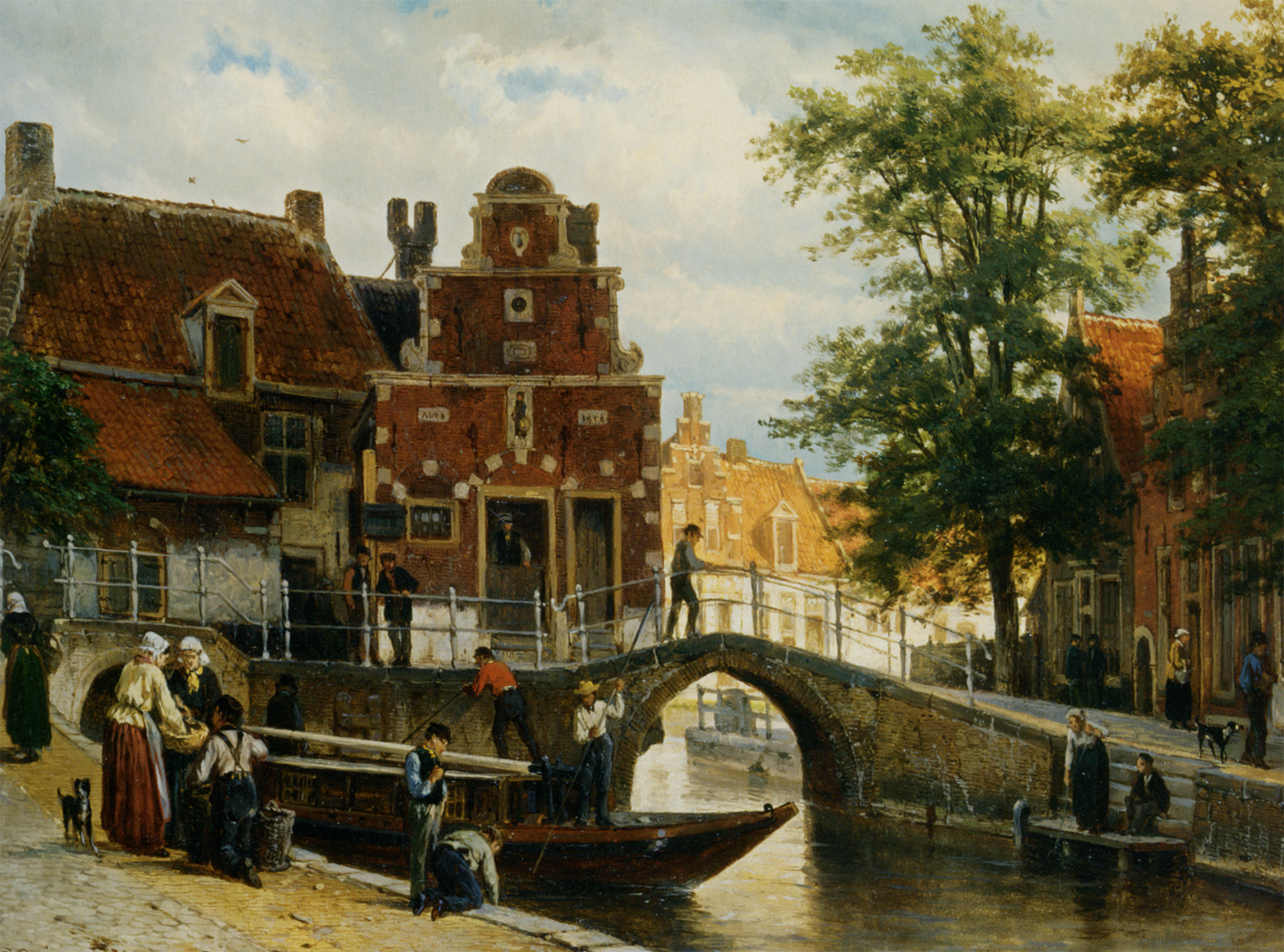This is a beautifully detailed painting of a small, likely historic European village set along a narrow river or canal, with emphasis on daily life activities. The village features old, somewhat decrepit brick buildings with slanted, tiled rooftops, some highlighted by sunlight pouring in from the background, giving the scene a warm, nostalgic atmosphere. In the center of the image, a stone walk bridge arches over the water, with one person crossing it. Below the bridge, a small boat navigates the stream, manned by two men—one in a white long-sleeve shirt, dark blue pants, and a cowboy-style hat, and the other possibly in an orange shirt. 

To the left of the painting, you see a large red-bricked building, and in the lower left, two women covered from head to toe in long dresses and white bonnets are standing with a small dog beside them. They are being observed by a boy in suspenders. Nearby, a child or another person is leaning over, perhaps picking something out of the water, while another man stands close by, looking down. The painting's palette includes dominant tones of blue, white, green, brown, and hints of red, creating a vibrant yet harmonious depiction of a lively village scene.